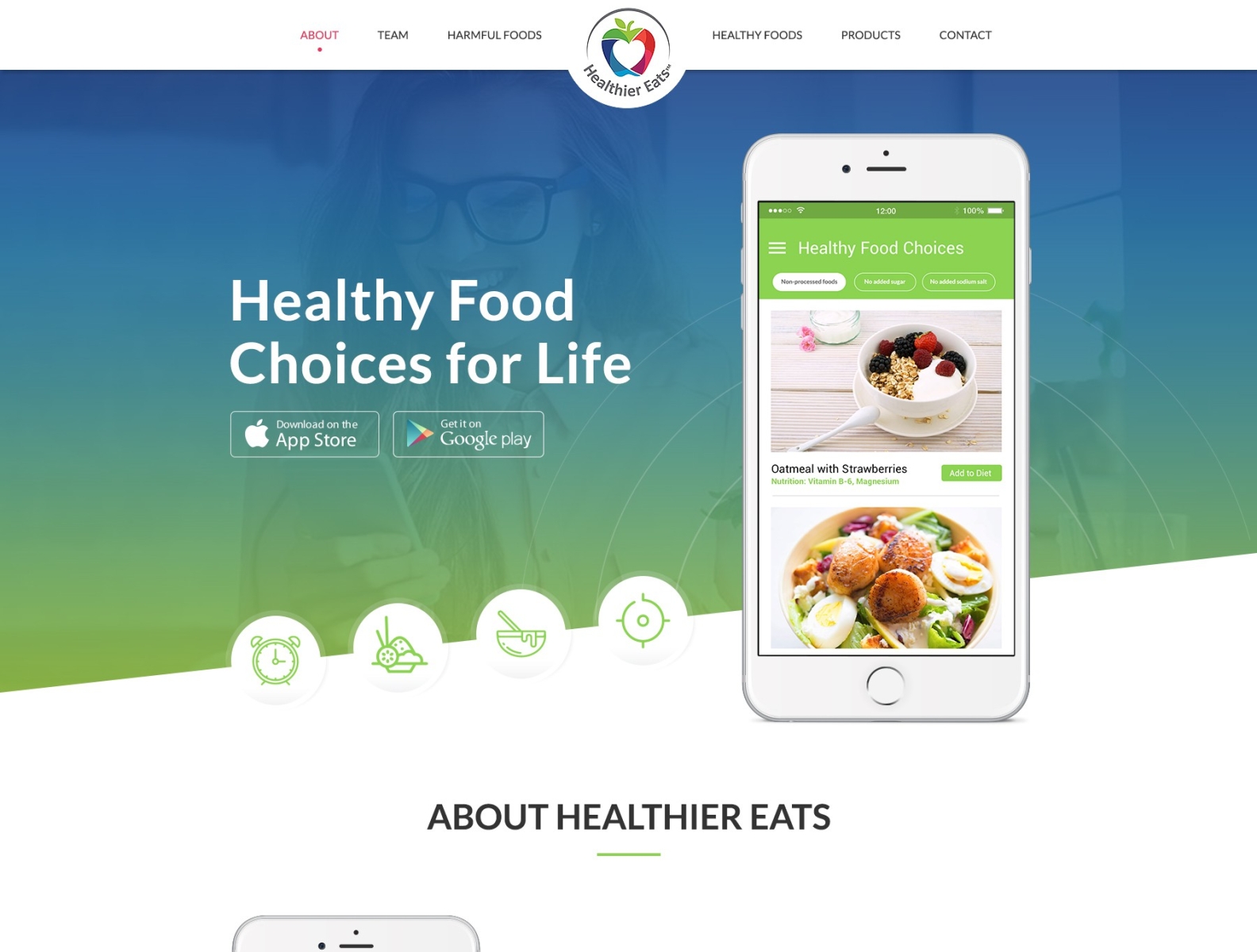The screenshot depicts a website focused on promoting healthy eating. The top header, set against a solid white background, features a navigation menu with buttons listed from left to right: About (in dark pink), Team, Harmful Foods, Healthy Foods, Products, and Contact. At the center of the header is a colorful apple logo with the text "Healthier Eats" beneath it.

Below the header, the background transitions into a muted blend of blue, green, and yellow hues. Dominating this section is a somewhat indistinct image of a young woman wearing glasses. Superimposed over her head is bold white text reading "Healthy Food Choices for Life."

Further down, the website offers two prominent buttons for downloading an app, one for the Apple App Store and the other for Google Play. To the right of these buttons, an image of a smartphone displays a screenshot of the Healthy Food Choices app, which showcases two appetizing dishes of healthy food.